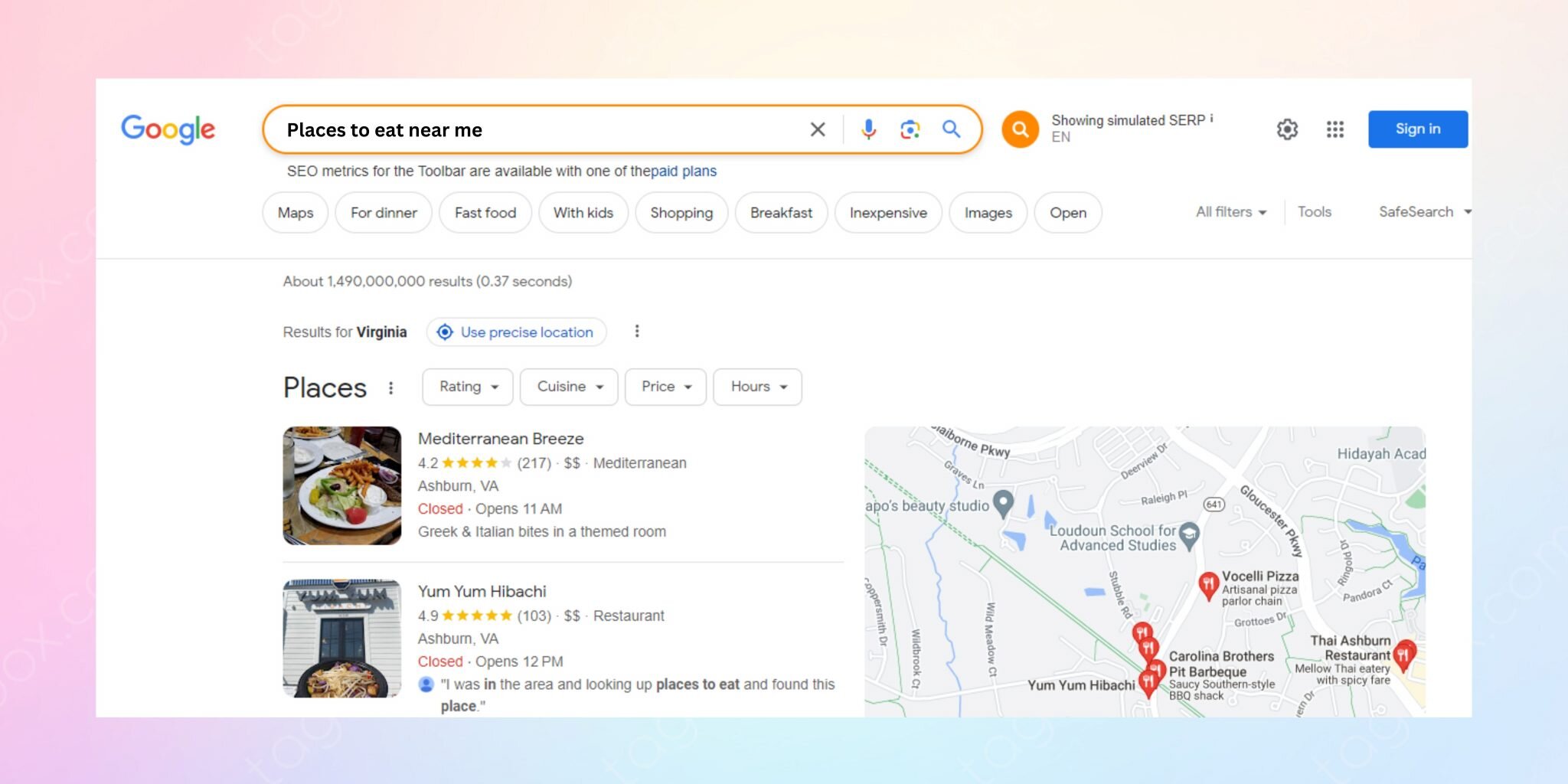This image is a digital composition featuring a screenshot superimposed onto a vibrant, gradient background card arranged in a landscape orientation. The background exhibits a rich tapestry of colors: starting from shades of pink blending into purple from the upper left to the lower left, transitioning from purple into blue from the bottom left to the bottom right, shifting from light blue into a creamy hue from the bottom right to the upper right, and finally looping back towards the upper left corner. 

The central focus is a screenshot of a Google search query "places to eat near me," prominently highlighted in orange with the text set in boldface. Below the search query, buttons offer various options such as maps, dinner, fast food, kids, shopping, breakfast, inexpensive, images, and open. A note next to the search button states "showing simulated SERP" (Search Engine Results Page). In the upper right corner, a "Sign in" button is visible. 

The search results displayed are for Virginia, featuring a precision location button and an initial listing of two places: Mediterranean Breeze and Yum Yum Hibachi. On the right side of the screenshot, a map populated with multiple dining locations provides a visual guide to the listed eateries.